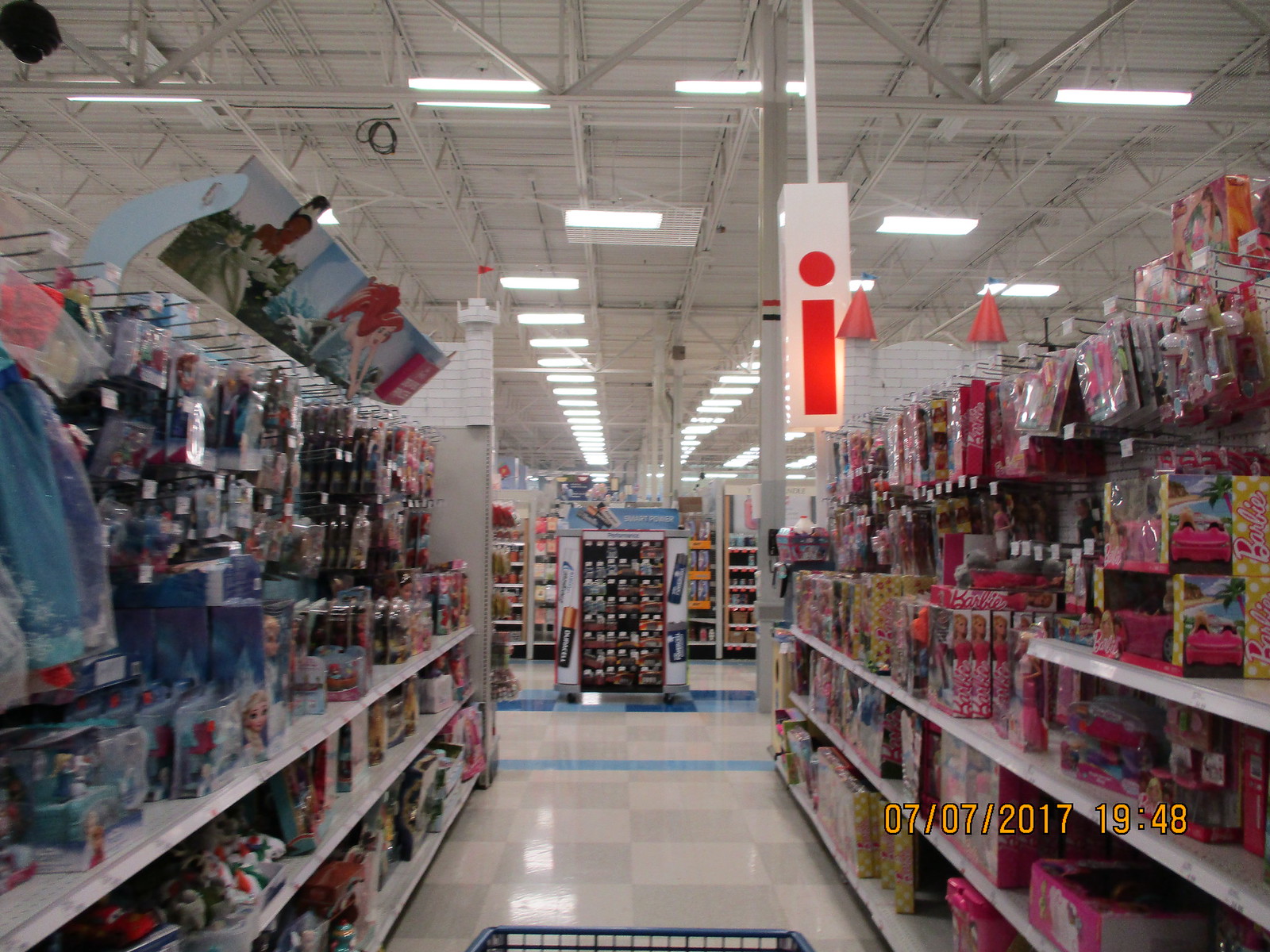In this photograph taken in the middle of a toy aisle in a store, the viewer's perspective from behind a blue shopping basket reveals a detailed scene. The floor is adorned with a white and gray checkered tile pattern, extending toward the end of the aisle where blue stripes run parallel. At the bottom right corner, a digital timestamp reads "07 07 2017 19:48," indicating the picture was likely taken with a point-and-shoot camera. The ceiling above is a bare metal roof, featuring numerous fluorescent light fixtures and metal support beams. 

On the left side of the aisle, the shelves are stocked with Little Mermaid toys, highlighted by a long sign displaying Disney princesses Tiana and Ariel. To the right, the shelves teem with Barbie merchandise, their packaging prominently displaying images of Barbies and bursts of pink color. A notable feature on this side is a large rectangular white plastic box on a pole, emitting light from a red eye-like fixture. 

Directly in the center of the background, a display of various batteries catches the eye, characterized by a white frame and blue top. Shelves stocked with indistinct merchandise flank this display. This comprehensive image captures the vibrant and organized chaos typical of a toy aisle in a large retail setting, blending elements from both sides to create a rich and detailed glimpse into the shopping experience.